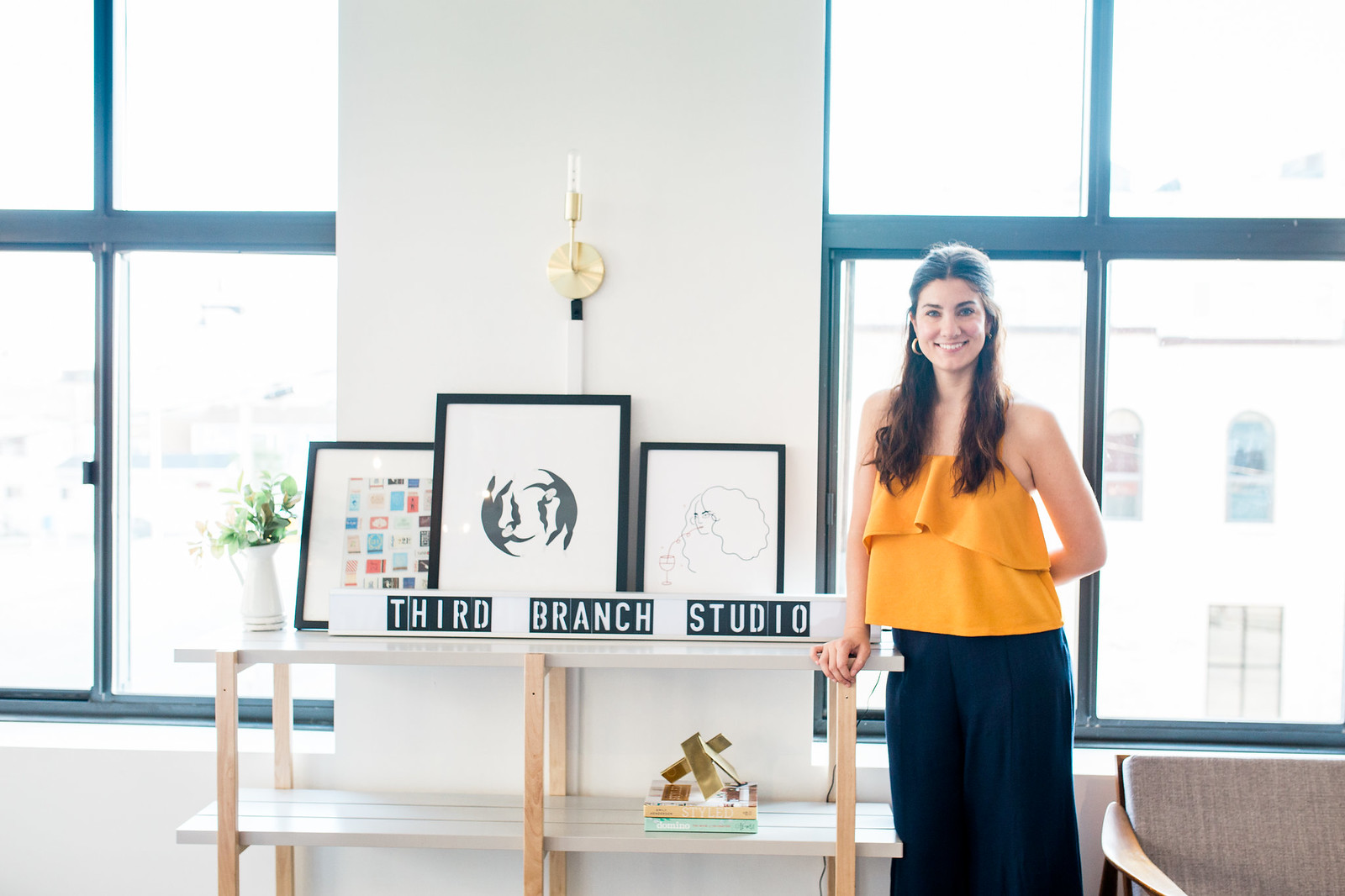The image captures a beautifully lit room with large rectangular glass windows making up the background, allowing ample natural light to flood in. There are at least eight windows, framing a small white wall section adorned with a white table-cum-shelf unit. This unit features light wooden legs, six in total, which connect two white shelves. On the top shelf sit three picture frames displaying different pieces of artwork: one resembling a collection of stamps, another showcasing a circular design, and a third sectioned into blocks with blue background and white letters that spell out "Third Branch Studio."

In front of this setup stands a smiling woman with long, brown hair styled to chest length, partly pulled up. She is wearing a bright yellow tank top and wide-leg, poofy blue pants. She appears to be the artist of "Third Branch Studio," posing confidently with her work. Her hand rests on the shelf, next to a small vase with green leaves on the opposite side, complementing the artistic display. A beige upholstered chair can be seen to the right side of the frame, adding a touch of coziness to the scene. The windows, with their blue frames, provide a scenic streetscape view, further enhancing the airy and creative atmosphere of the room.